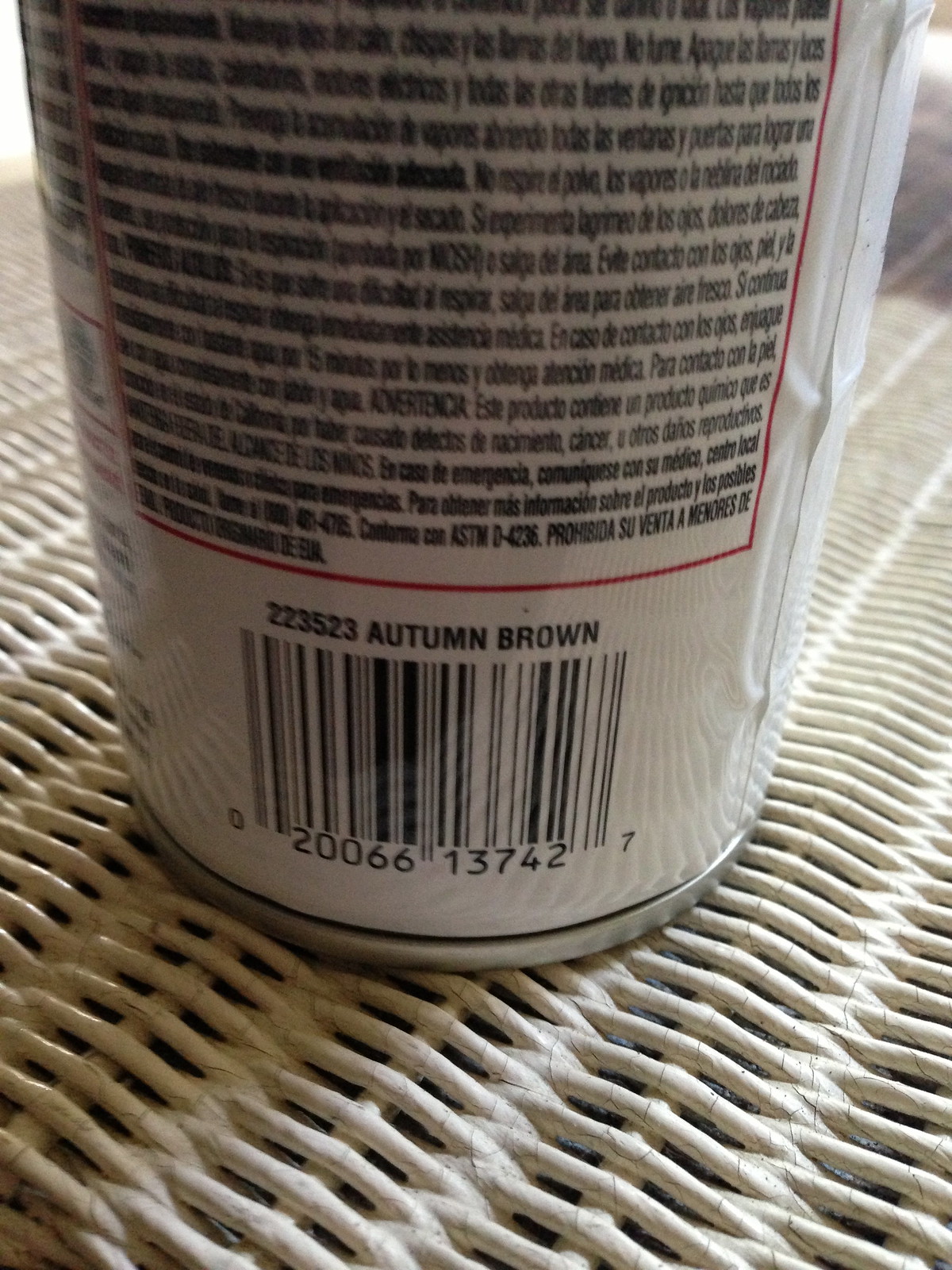This image depicts a can with extensive Spanish text, although the image is slightly blurry, making the text difficult to read. The prominent feature is a large black paragraph of text encased in a red border, accompanied by additional but less legible writing to its left at the edge of the can. Near the bottom, there is a scannable label with printed numbers "223523" and "Autumn Brown," suggesting it may be a spray paint can. Beneath this label, another sequence of numbers, "020066137427," is visible. The can rests on a wicker-like surface composed of white interconnecting sticks.